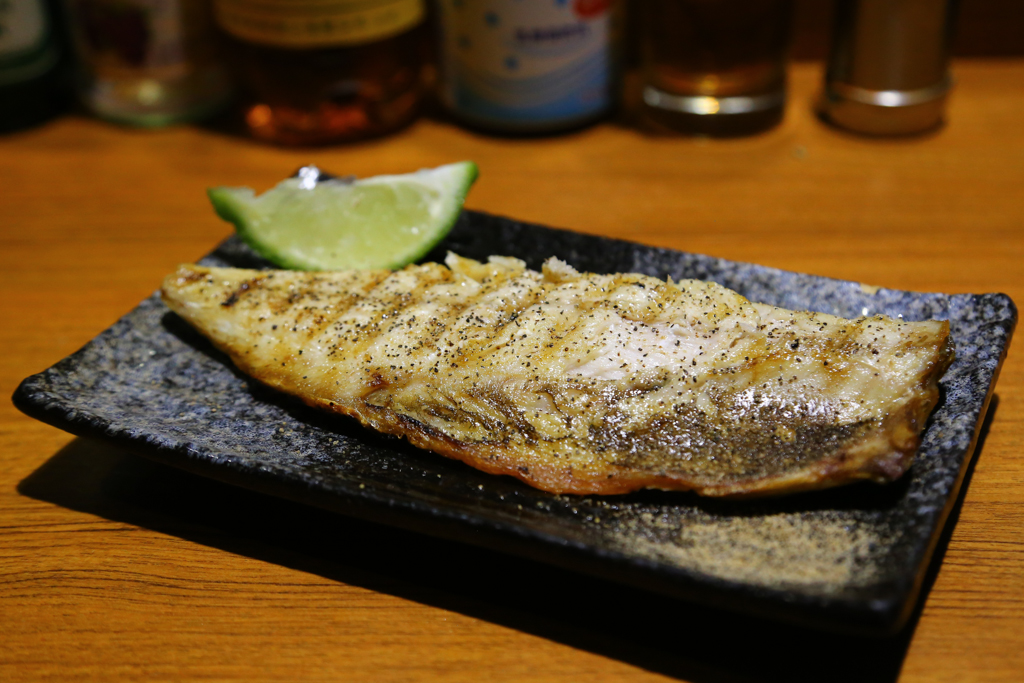This detailed photograph captures a beautifully grilled fish fillet, generously seasoned with black pepper, centrally positioned on a decorative, black, rectangular platter with a pebble finish. The fish, displayed prominent with its golden crust and tapering shape, suggests the tail was on the left. Accompanied by a vibrant green lime wedge on the top left, the dish contrasts elegantly against a honey-golden oak wooden table, enhanced by good lighting. In the blurred background, several condiment and drink bottles add depth and context, enhancing the indoor restaurant setting's ambiance. The image reflects a sophisticated instance of food photography, focusing on realism and representationalism.